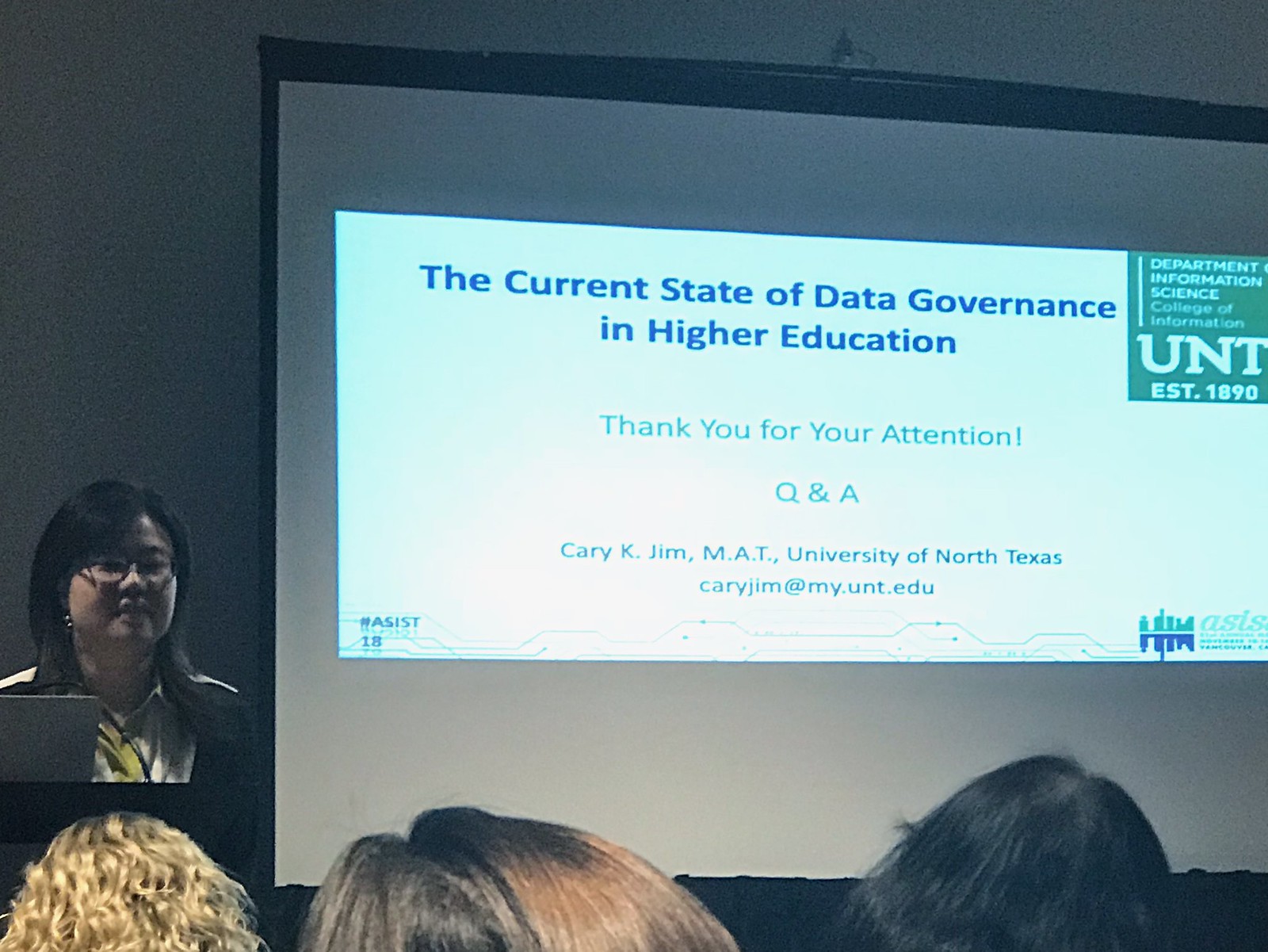In the photograph, an Asian woman with glasses stands at a podium next to a laptop, delivering a presentation on "The Current State of Data Governance in Higher Education." She is positioned on the left side of the frame, and the image is cut off at her waist. She has long black hair and is wearing a light-colored shirt. The setting appears to be a dark room to enhance the visibility of the projected slide. The projection screen dominates the image, displaying the slide in predominantly blue and green text, with important details such as "The Current State of Data Governance in Higher Education," followed by "Thank you for your attention, Q&A," presented by Carrie K. Kim, MAT, from the University of North Texas. Her email is listed for further queries. The upper right corner of the slide states "Department of Information Science, College of Information, UNT," and the bottom left corner shows "ASSIST, number 18." In the foreground, the tops of three attendees' heads, with varying hair colors—blonde, brown, and dark—are barely visible, indicating an audience.